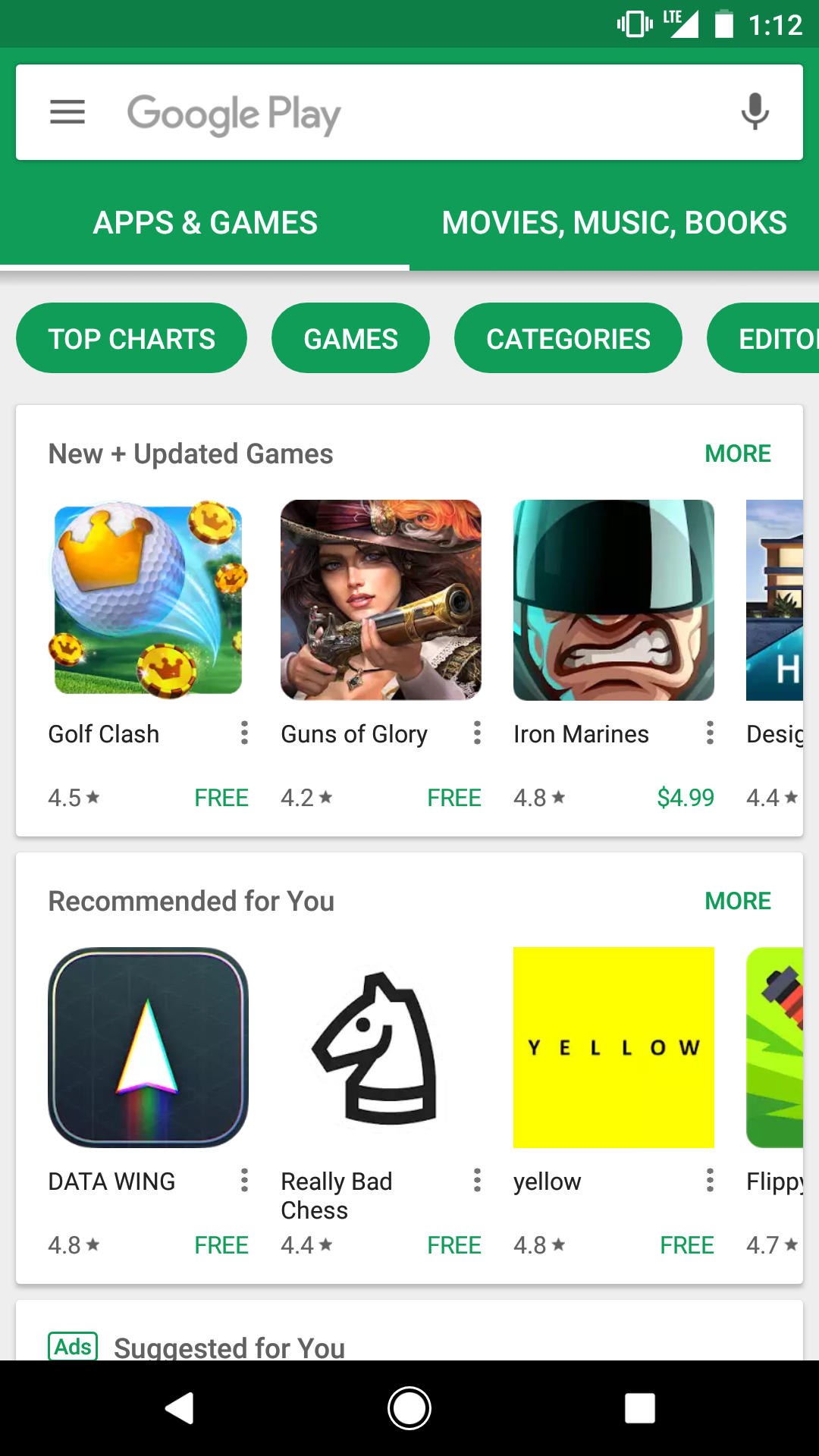The screenshot captures the interface of the Google Play Store app displayed on an Android mobile device, as identified by the navigation buttons at the bottom of the screen—a left-pointing arrow for the back button, a circle for the home button, and a square for recent apps—all positioned on a black banner. 

The primary focus of the screenshot is the Google Play Store, distinguished by its dominant green theme. At the top is a green header containing a white, rectangular search box with a Google Play icon, accompanied by a microphone icon for voice search. Below this green section, white text categorizes content into "Apps & Games," "Movies," "Music," and "Books." The "Apps & Games" section is highlighted, indicated by an underline.

Further down, several buttons refine the search results: "Top Charts," "Games," "Categories," and "Editor's Choice." Below these buttons, a selection of game thumbnails is visible, showcasing titles such as "Golf Clash," "Guns of Glory," and "Iron Marines," characterized by vibrant, cartoonish graphics.

Beneath this featured game section is the "Recommended for You" area, presenting additional game thumbnails based on the user's preferences. The previous list of games is categorized under "New and Updated Games."